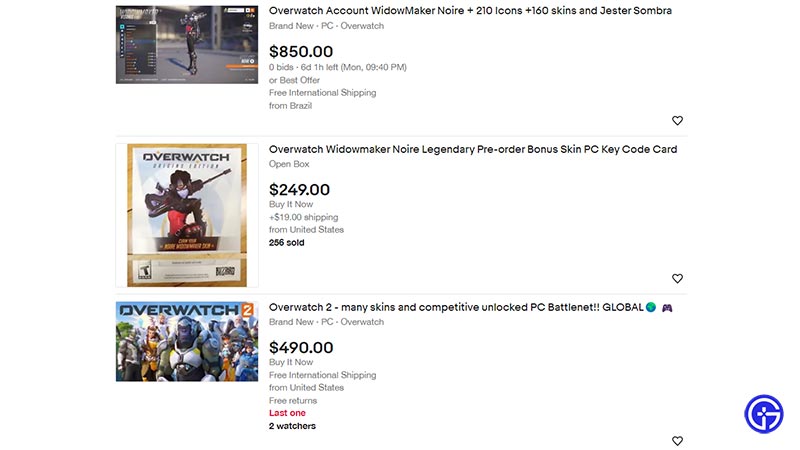Screenshot of a marketplace for Overwatch items and accounts:
The top listing features an Overwatch account that includes the coveted Widowmaker Nair with 210 icons, 166+ skins, and a Jester Sombra skin, priced at $850. The listing has no bids with 6 days and 1 hour remaining, and offers the best offer option with free expedited shipping from Brazil. Another notable item is a Legendary pre-order bonus skin for Widowmaker, available as a PC code card for $249 or a buy-it-now option for $256 (with $19 shipping) from the United States. Additionally, there is an Overwatch 2 account with numerous skins and competitive unlocks, available for $490 with free international shipping and free returns from the United States. This last item is indicated as the last one with two launches mentioned. The webpage appears to be dedicated to the sale of Overwatch digital goods and accounts.